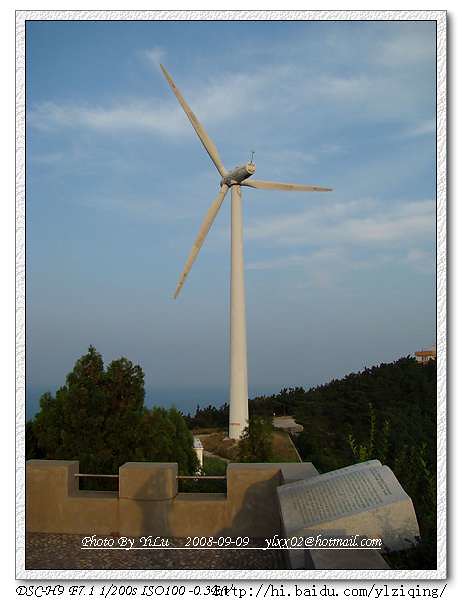In the image, the vast majority of the upper section is filled with a vibrant blue sky dotted with wispy white clouds, indicating it's daytime. Dominating the center of the picture is a large white windmill, which extends from the middle to the upper third of the frame. This windmill has three sharp, pointed blades, reminiscent of an airplane propeller, and it is likely made of metal. Below the windmill, the landscape features lush green bushes and trees, climbing up what appears to be a small hill or mountain. At the crest of this hill sits a tiny house, dwarfed by its surroundings.

On the left side of the scene, a variety of trees add to the verdant setting. Additionally, there is a concrete walkway adorned with poles that serve as a barrier, suggesting a scenic overlook or memorial area. In the bottom right corner of the image, a stone slab is visible, possibly containing descriptive information about the site. Finally, white text reads: "Photo by Yilu, 2008-09-09," followed by an email address, "yhxx02@hotmail.com," and an accompanying website link.